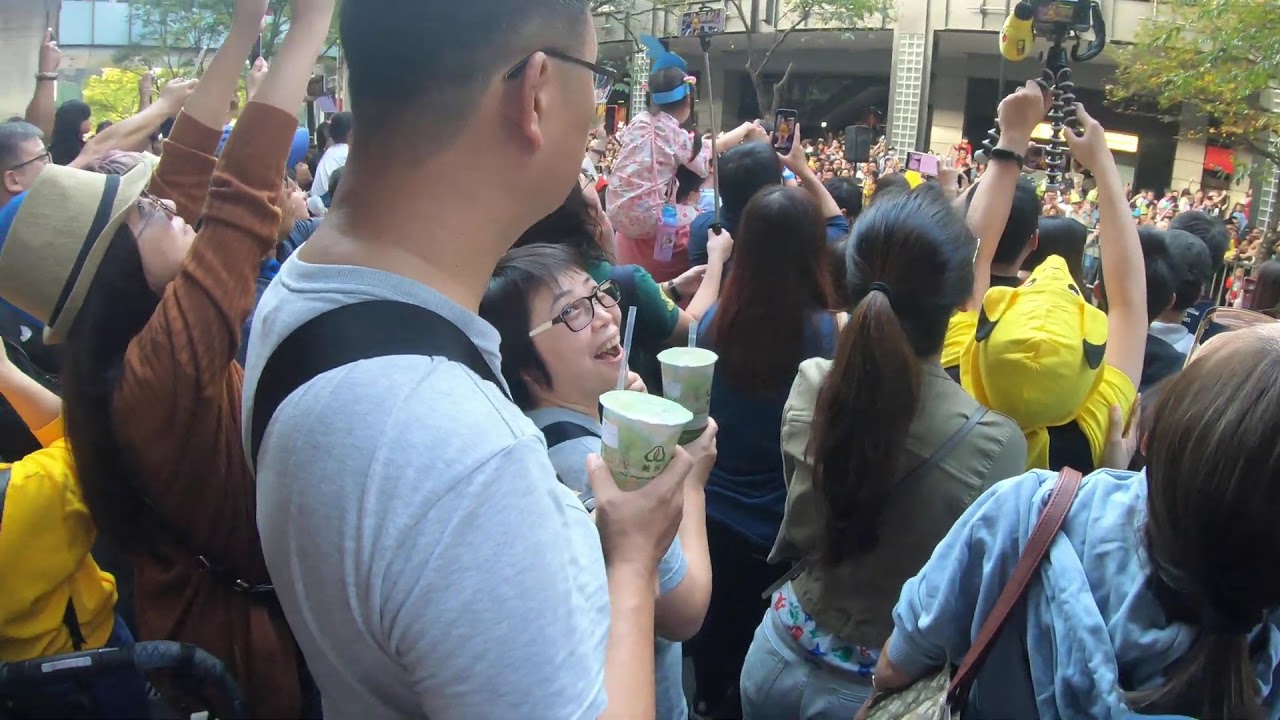This photorealistic image captures a densely packed crowd of predominantly Asian individuals standing outdoors in front of a large gray building, suggesting an event like a parade. People are standing shoulder to shoulder, mostly turned in the same direction, engrossed in the scene ahead. The crowd includes individuals with various hair colors and styles, many with dark hair, some adorned in costumes. The focal point of the image is a man upfront facing the direction of the event; he has short hair, glasses, a blue shirt, and is holding a green drink with a straw. Next to him, a woman with short dark hair and glasses, also holding a green drink, is partially turned towards the camera, smiling. Around them, several attendees are capturing the moment with raised phones, selfie sticks, and tripods. In the background, more people are visible beyond the crowd and trees with green leaves, hinting at some central activity between these groups. A child is seen perched on an adult's shoulders, while someone in a yellow costume with ears and a nose holds a tripod high above their head. This vibrant assembly conveys the excitement and anticipation felt by the crowd.